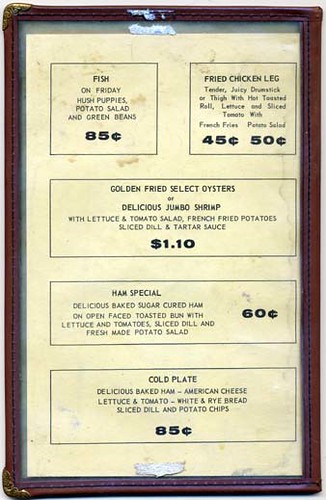The image displays a beautifully framed vintage menu, encased in a simple yet elegant brown frame. The menu is presented on a white background, with multiple small black boxes featuring black text, detailing various delectable offerings and their prices.

1. **Fish on Friday**: For just $0.85, customers could enjoy a meal consisting of fish, hush puppies, potato salad, and green beans.

2. **Fried Chicken Leg**: This option included a tender, juicy drumstick or thigh served with a hot tossed roll, fresh lettuce and sliced tomato, paired with either french fries or potato salad, priced between $0.45 to $0.50.

3. At the center of the menu:
   - **Golden Fried Select Oysters or Delicious Jumbo Shrimp**: This special dish, sold for $1.10, was served with lettuce and tomato salad, french fried potatoes, a sliced roll, and tartar sauce.

4. **Ham Special**: For $0.60, patrons could savor delicious baked sugar-cured ham on an open-faced toasted bun, accompanied by lettuce, tomato, a sliced dill pickle, and freshly made potato salad.

5. **Cold Plate**: This option, at $0.85, offered a delightful combination of baked ham, American cheese, lettuce, tomato, both white and brown bread, a sliced dill pickle, and potato chips.

The detailed menu is a nostalgic glimpse into classic culinary offerings and their remarkably economical prices.